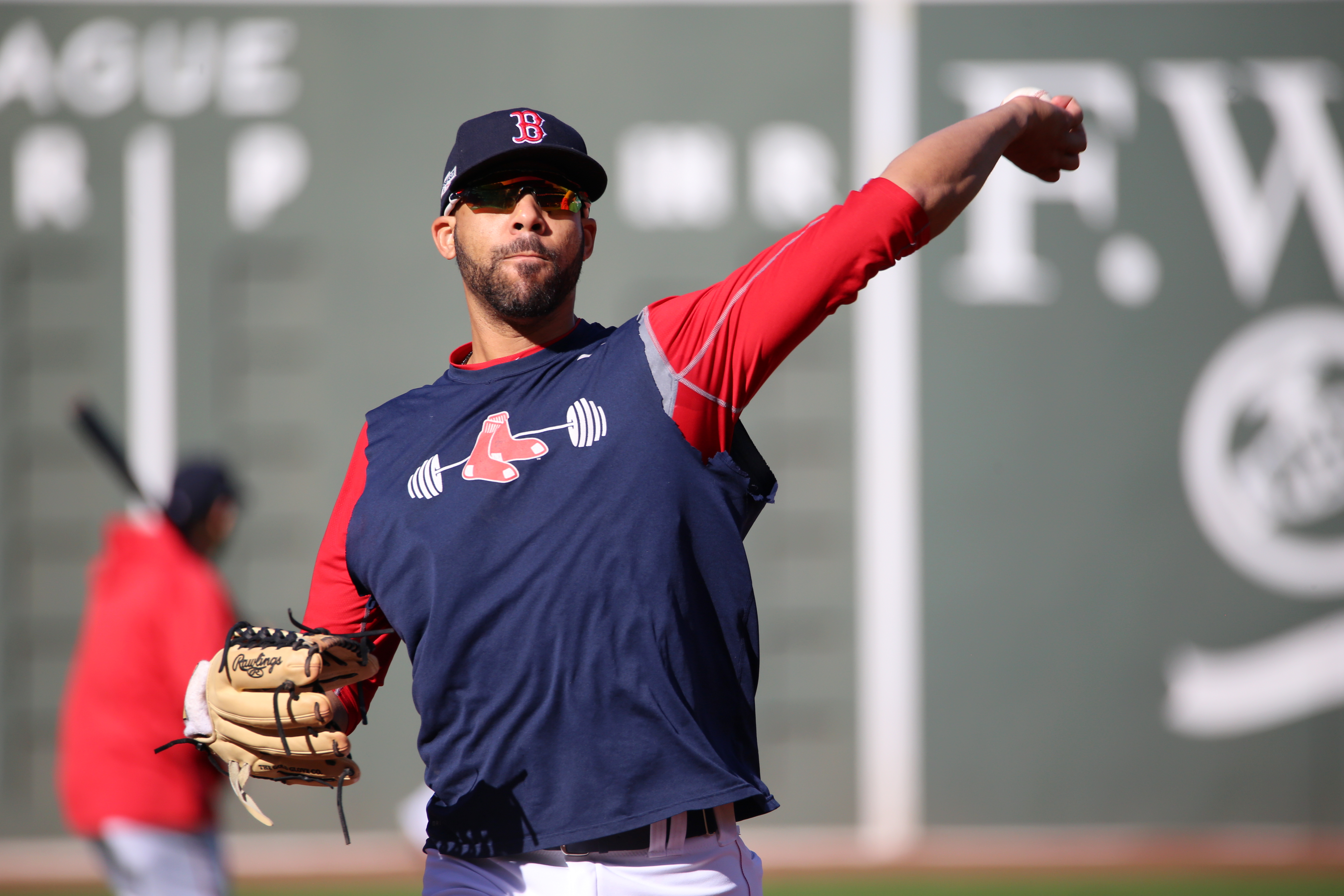This outdoor daytime photograph, rectangular in shape (approximately six inches wide by four inches tall), features a man in a baseball uniform positioned just left of center, captured from the hips up. The man has light brown skin and a closely trimmed beard and mustache. He is wearing a navy blue baseball cap adorned with a red 'B' bordered in white, suggesting it represents the Boston Red Sox. His uniform includes a red long-sleeved shirt visible at the collar and cuffs underneath a navy blue sleeveless shirt with jagged edges. The sleeveless shirt features a striking graphic of a long barbell with weights and a pair of red socks at its center.

His left arm is dramatically twisted backward, poised to throw a baseball that is visible in his hand, while his right arm, bent at the elbow, wields a catcher's mitt. His white pants are just visible at his hips. The image background is dominated by a large, blurred wall with some indistinguishable white lettering. In the lower left corner, another player in a red shirt and white pants is visible, also blurred, holding a baseball bat and preparing to hit. This detailed scene vividly captures the intensity and motion of the pitcher mid-throw.